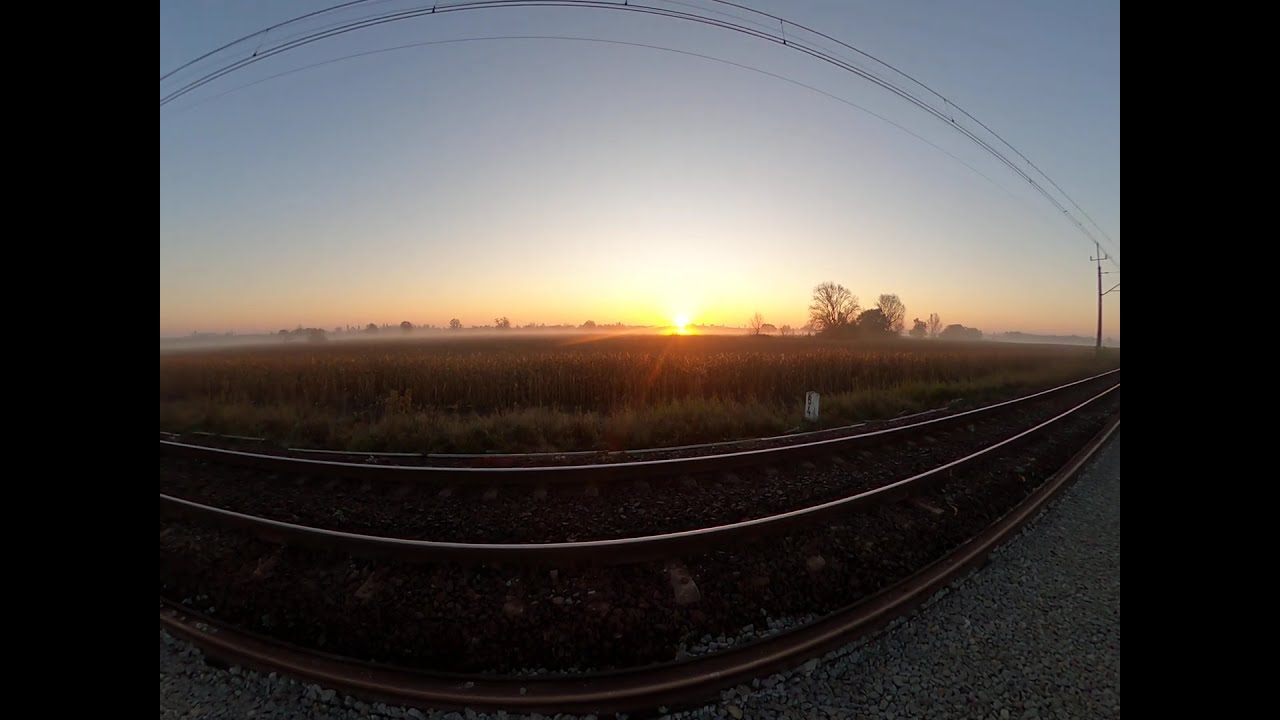This panoramic photograph captures a serene outdoor landscape at sunset. Dominated by a vast, empty field of crops, possibly corn, the scene is framed by a distinct black band on the left and right sides, adding a finishing touch to the image. The bright yellow sun is setting above the horizon, casting a warm blend of orange and pink hues across the clear sky. In the distance, a tree line forms the boundary of the field, while a few indistinct buildings are visible, adding a touch of human presence to the natural beauty. In the foreground, a set of three railroad tracks stretches across, surrounded by typical gray gravel. The setup includes metal tracks and a darker gravel area, providing an interesting contrast to the lushness of the field. To the right, a telephone pole and scattered electrical wires cross the scene, subtly breaking the rustic tranquility. Overall, the photograph effortlessly merges elements of industrial and natural beauty, encapsulating a tranquil moment at dusk.